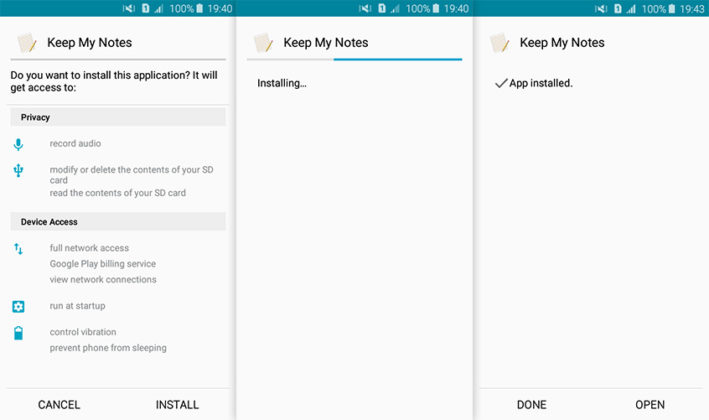Here is a cleaned-up and detailed caption for the given image:

---

Three tiled side-by-side phone screenshots detail the installation process of the "Keep My Notes" application. 

**Screenshot 1 (Left):** Displaying a blue taskbar at the top, the phone screen shows that it is on silent mode, with 3 out of 4 signal bars, a 100% battery level, and the time at 7:40 PM. In the main view, an installation page for "Keep My Notes" is open. At the center, two yellow sticky notes are diagonally positioned, overlapping. The page outlines the app's privacy permissions, including recording audio, modifying or deleting the contents of the SD card, and reading the contents of the SD card. To the left, icons representing a teal microphone and a three-prong USB logo appear. Below, under "Device Access," there are permissions for full network access, Google Play billing service, and viewing network connections, denoted by teal up and down arrows. Further permissions listed include the ability to run at startup, control vibration, and prevent the phone from sleeping, each represented with respective teal icons: a white gear and a battery indicator. The screen features two options at the bottom: "Cancel" and "Install."

**Screenshot 2 (Middle):** The time remains 7:40 PM, and the screen shows the ongoing installation process of "Keep My Notes." A black background with a teal progress bar indicates that the app is currently installing. Notably, the text "Keep My Notes" is displayed alongside a checkmark confirming the app installation. At the bottom of the screen, two buttons labeled "Done" and "Open" are visible, signifying the completion of the installation process.

---

This version provides a structured and detailed description of each screenshot, improving clarity and readability.